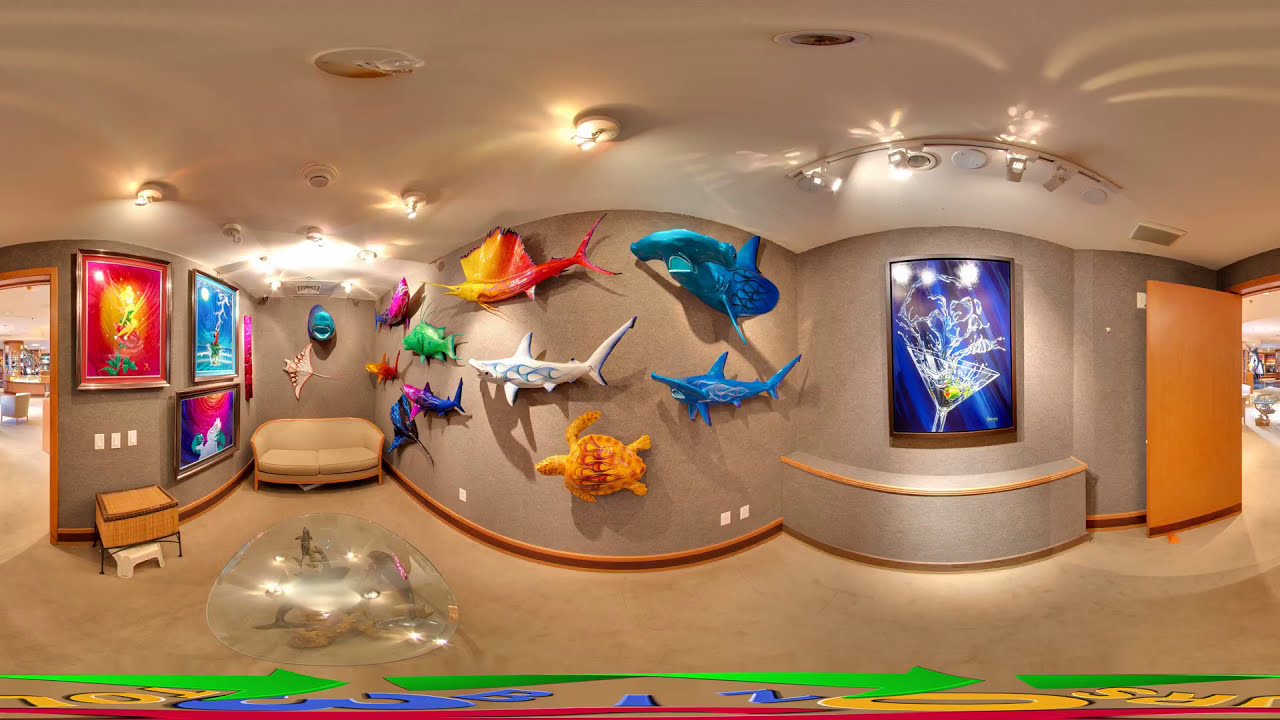This photograph captures the interior of a museum gallery, an art exhibit with a distinctive underwater theme. The walls are adorned with a vibrant collection of sea creature sculptures, including a variety of fish, turtles, sharks, a ray, and a sailfish, all painted in multicolored and unnatural hues like turquoise, white, red, blue, green, orange, yellow, and purple. These sculptures appear to be made of plastic and are mounted against a backdrop of light brown and gray fabric walls.

The image is taken with a wide-angle lens, creating a slightly distorted fisheye view of the room. The ceiling is white and fitted with numerous spotlights that illuminate the detailed artwork. On the small right wall, there's a large poster featuring a martini with its content spilling out, set against a blue background with a black frame. Below this, a light brown wooden door stands open, revealing an extension of the exhibit area.

To the left side of the image, additional paintings are visible, including depictions of sea life, Tinkerbell, and Ursula from The Little Mermaid. There's also a beige couch situated there and another doorway leading further into the gallery. The letters "R," "S," and "O" appear at the bottom of the photograph, along with some green arrows. Inside the room, various lighting fixtures cast beams on the portraits and sculptures, enhancing the vibrant and dynamic atmosphere of this museum space.